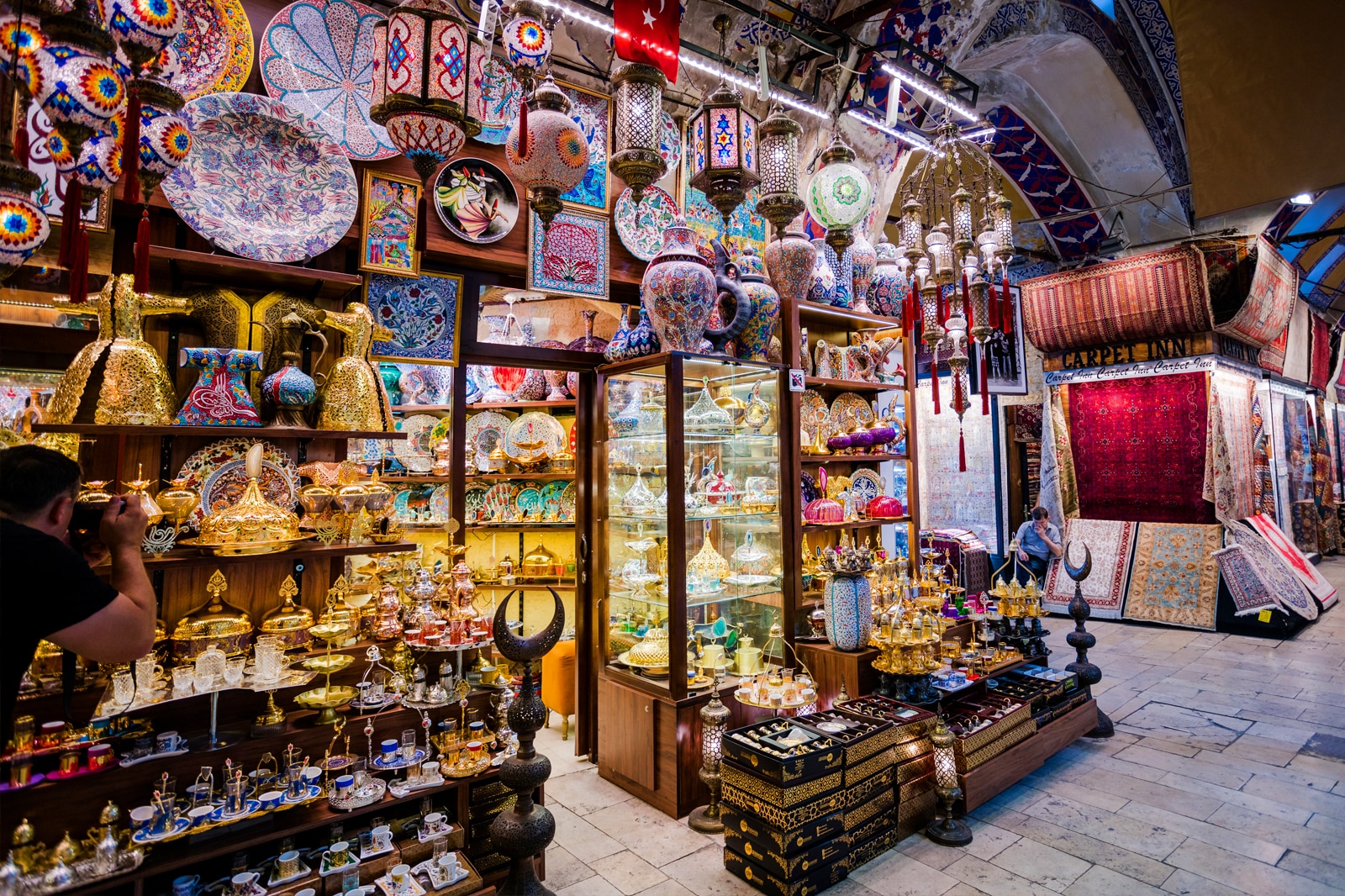This photograph captures a bustling indoor Indian bazaar set inside an old building with a tan ceiling. The focal point is a shop displaying a variety of ceramic dishes and glassware with intricate designs. Among the items, there are numerous vases and gold trinkets on shelves, suggesting they are quite valuable. On the left side, a man in a black t-shirt is leaning down to take a photo of the gold items with a camera. The shelves also feature colorful metal and glass statues, including hues of blue, purple, pink, yellow, and gold. A flag with a red background and a white star is displayed prominently. 

On the right side of the walkway, another shop showcases an array of oriental or Indian-style rugs and fabrics, some laid out on the ground and others hanging from the shop. The bazaar is adorned with various large plates on the walls, characterized by vibrant colors like pink, purple, blue, yellow, and green. One remarkable white plate above a doorway is decorated with violet and red floral designs. 

Beneath the doorway with blue, white, and red designs, the floor consists of white, tan, and black or grayish brick or stone. Towards the left, there's a crescent moon-shaped black statue atop some boxes, possibly gold and black, with a brown shell in front. The scene is vibrant and full of intricate details, reflecting the rich and colorful atmosphere of an Indian market.